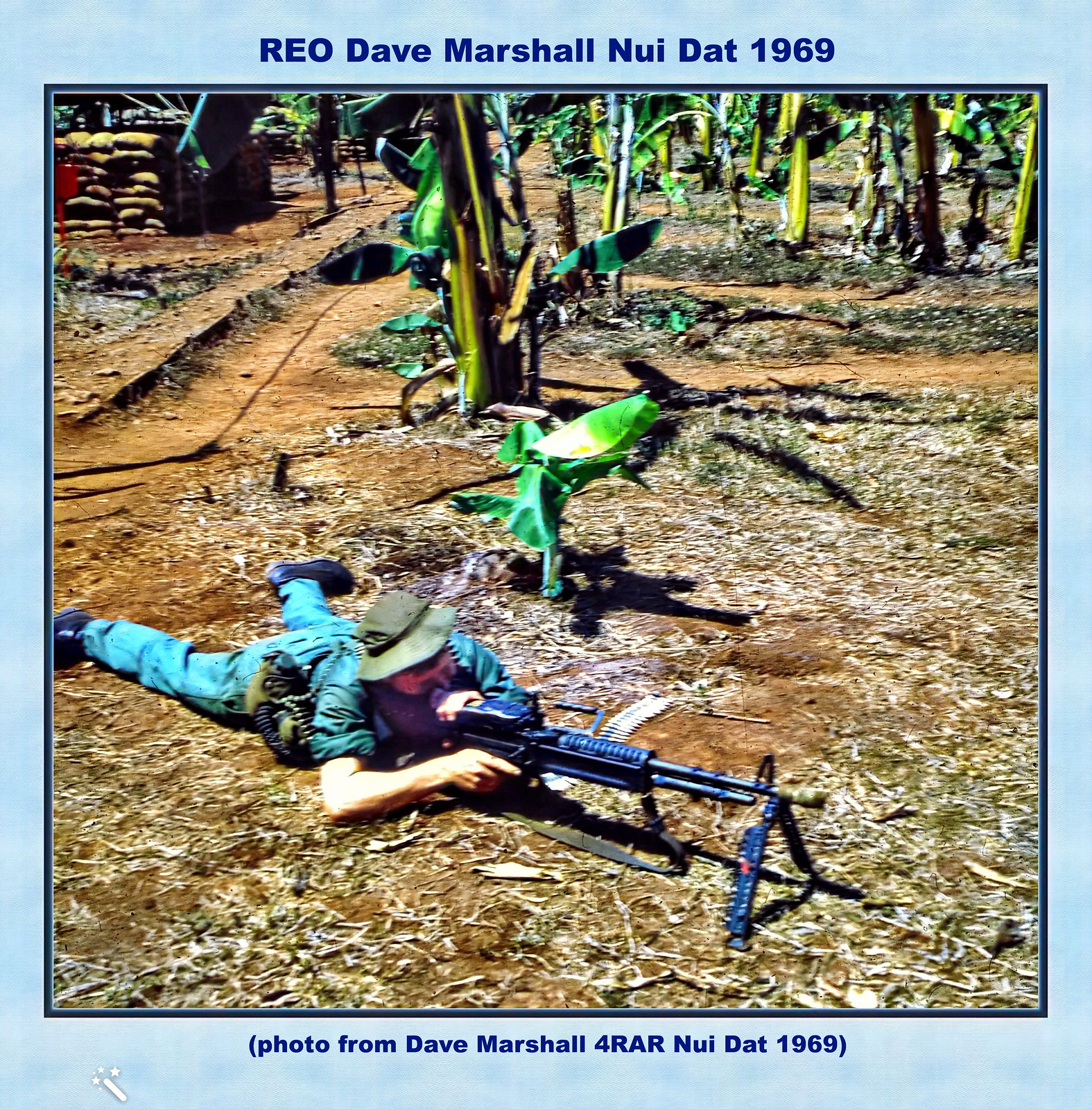This appears to be a photograph from the Vietnam War, formatted like a postcard with a light blue border and blue text. The caption at the top reads, "REO Dave Marshall Nui Dat 1969," while the bottom text states, "Photo from Dave Marshall for RAR Nui Dat 1969." The image shows a soldier lying on the jungle floor, potentially during the Vietnam War. He is dressed in a green bucket hat, rolled-up sleeves, and blue jeans or pants. The soldier is positioned with a machine gun or rifle, which is mounted on a stand that elevates the nozzle above the ground. The scene includes a partially-cleared jungle area with visible forest plants and what appears to be a makeshift bunker or stacked sacks in the background. Additionally, there is a small dug-out trail near the soldier, adding to the wartime setting.